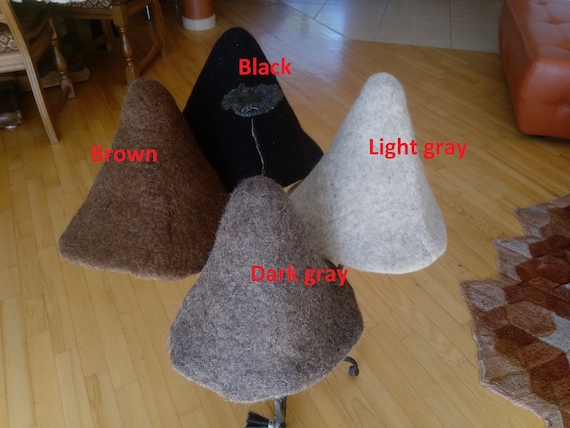This detailed color photograph captures a close-up of four conical fabric caps, arranged on what seems to be a rolling chair mechanism set on a light beige, planked wooden floor. The caps, reminiscent of dunce caps with rounded tops, are each uniquely colored and labeled in red lettering near their tops. The cap in the foreground is dark gray and labeled "Dark Gray," while to its right is a light gray cap labeled "Light Gray." On the left of the dark gray cap is a brown cap labeled "Brown," and the black cap in the background is labeled "Black." The scene reveals additional details including a patterned brown and gray rug with serrated edges in the bottom right, a glimpse of an orange-brown couch and a brown ottoman. The upper part of the photograph shows wooden chairs and a table positioned on what appears to be a white tile floor in the distance.